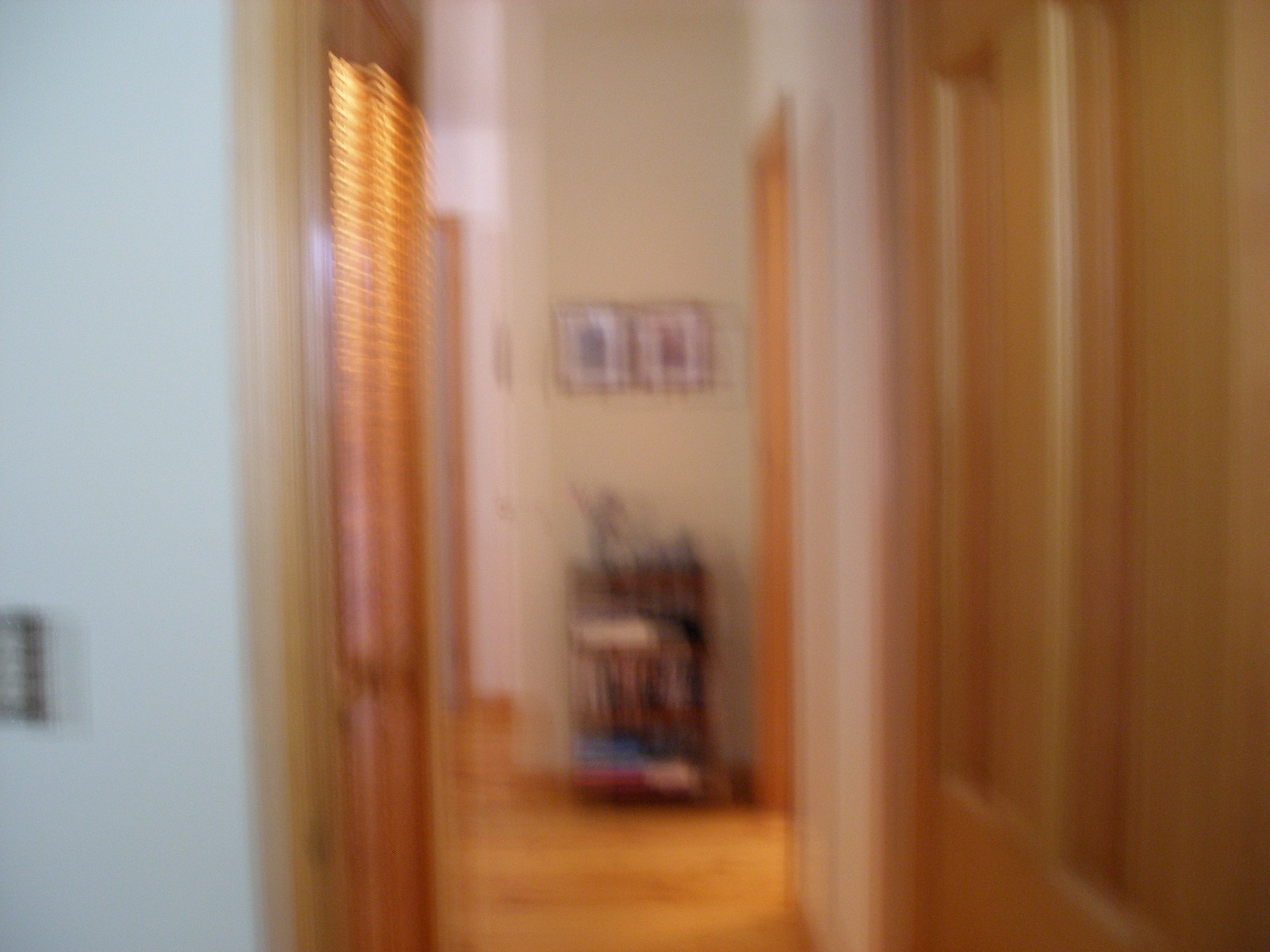This color photograph is highly blurry, making intricate details difficult to discern. The viewpoint seems to be from a doorway, looking into a room. On the left-hand side, there is a bluish-grey wall featuring a small black object that appears to be a light socket. To the right, a light brown, golden-colored door with panels is visible. A light source situated to the left of the scene casts illumination into the room. Between the hallway and the room, horizontal lines resembling blinds can be seen. The room features a wooden floor and light beige walls, contributing to its warm and inviting atmosphere.

Inside the room, another doorway on the right is slightly visible. On the left-hand side of the visible interior, two framed pictures are mounted on the wall. These frames are dark with white centers, each containing two smaller images inside them. A small shelving unit is placed within the room, possibly holding a plant on its top shelf and some books on the lower ones. Despite the blurriness, the arrangement hints at a cozy, well-decorated space.